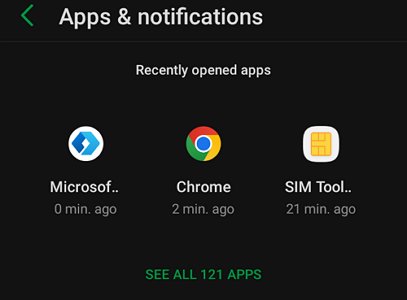This image is a screenshot of a phone interface, featuring a black background. The screen is divided into two main sections: a top bar and a primary display section below it. The top bar contains a green left-pointing arrow next to the text "Apps and Notifications" in white font. 

The main display area is labeled "Recently Opened Apps" at the top, also in white font. Below this header, there are three listed apps, each with an icon and a timestamp. On the left, there is a white icon with a blue diamond design, labeled "Microsoft," with the note "0 minutes ago" in white text. In the center, a familiar Chrome browser icon appears, followed by the text "Chrome, 2 minutes ago." To the right, there is an icon of a microchip in a goldish-yellow color set against a white background, labeled "SimTool," with the timestamp "21 minutes ago." At the very bottom of the screen, in a lighter grey font, is the option "See all 121 apps."